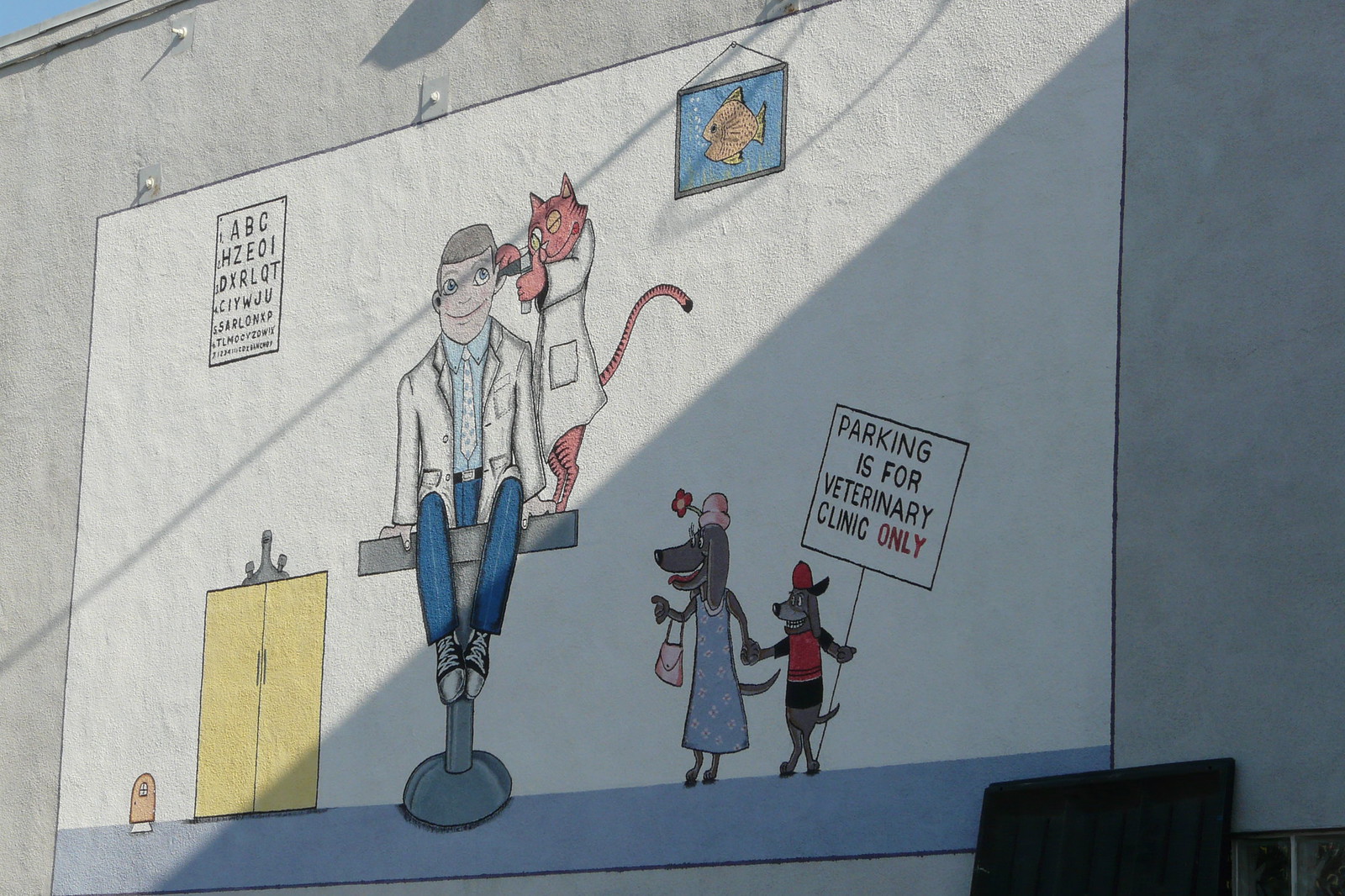The mural depicted in the image is painted on a large white section of a gray wall, showcasing a vibrant, sunlit scene. At the center of the mural, a whimsical cat, dressed in a doctor’s coat, attentively inspects a man's ear as he sits on an examination table, clad in blue pants, a white shirt, and a blue tie. On the left side of the mural, there is a detailed eye chart, complete with rows of randomized letters, indicating a vision test area. Below this, a drawn cabinet with a medical device perched on top adds to the clinic's setting. 

The bottom of the mural features a charming depiction of two dogs. One, a mother dog wearing a pink hat adorned with a flower and carrying a handbag, stands next to her smaller pup, who holds a sign proclaiming, "Parking is for veterinary clinic only." The top right of the mural is adorned with a picture frame containing an image of a goldfish swimming, adding a splash of aquatic color to the scene. 

Overall, the bright and clear setting of the mural, with sunlight casting shadows across its surface, brings this playful and detailed veterinary-themed artwork to life.